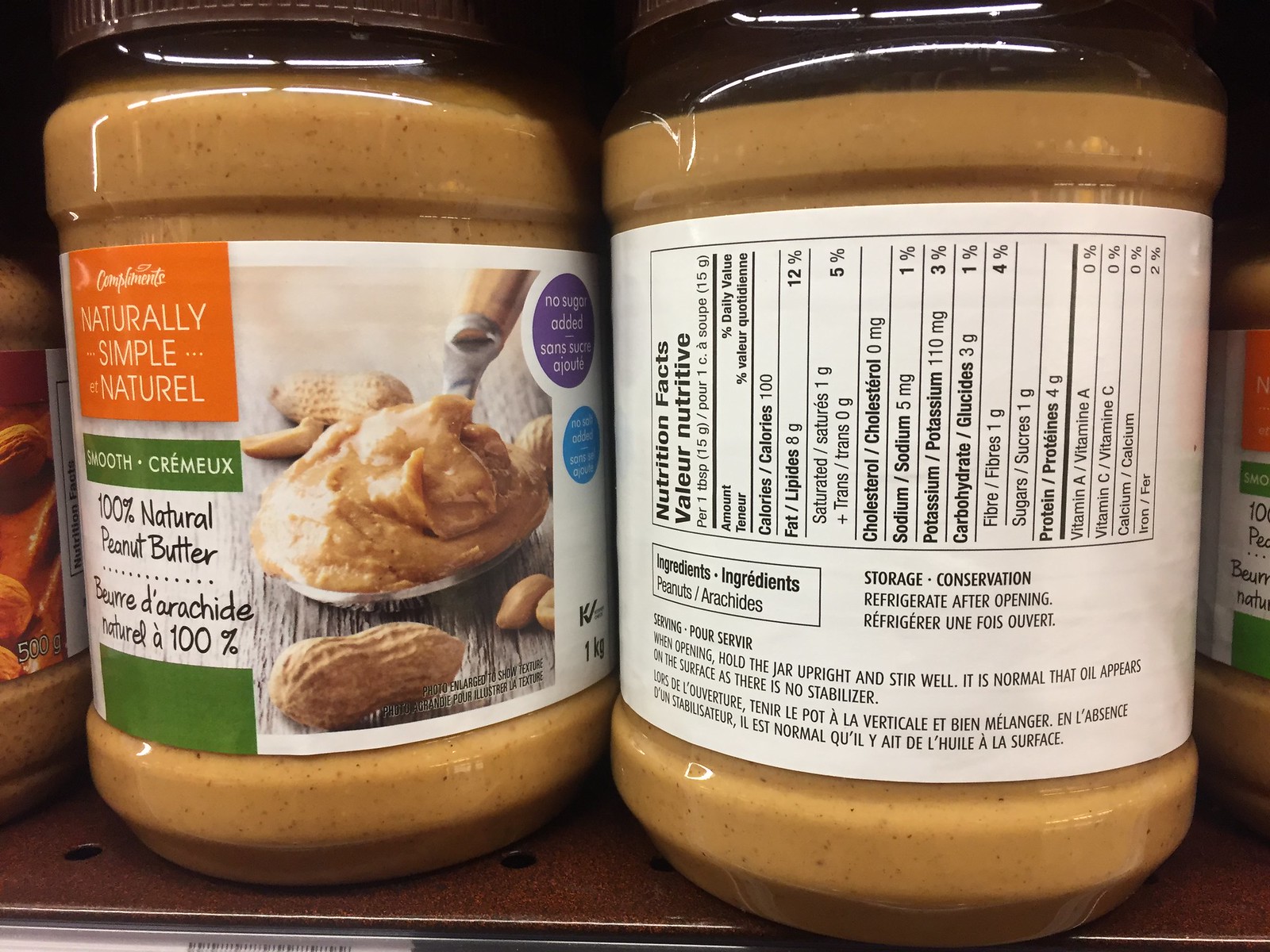The photograph captures a detailed, close-up view of two peanut butter jars on a perforated metallic grocery store shelf, likely in a Canadian supermarket where English and French are commonly spoken. The jars are in clear plastic containers, allowing the contents to be visible. The jar on the left prominently displays its front label, which includes an orange triangle in the upper left corner and the text "Naturally Simple Natural Smooth," along with the phrase "100% Natural Peanut Butter." The label also features a spoon scooping peanut butter, surrounded by images of shelled and unshelled peanuts, and states "No Sugar Added." Below this, there is a non-English word, possibly French, offering a bilingual labeling as seen commonly in Canada.

The jar on the right is turned 180 degrees, showing the nutritional information on its back label, which is mostly in French. It highlights the product's health attributes and includes an ingredient list and storage instructions. An obscure, partially visible strip at the bottom left corner of the photograph appears to be the product’s price label on the shelf, barely showing the top of a barcode.

This meticulous framing provides a comprehensive view of both the branding details and the nutritional information of the peanut butter, emphasizing the packaging design, bilingual labeling, and health-conscious branding.